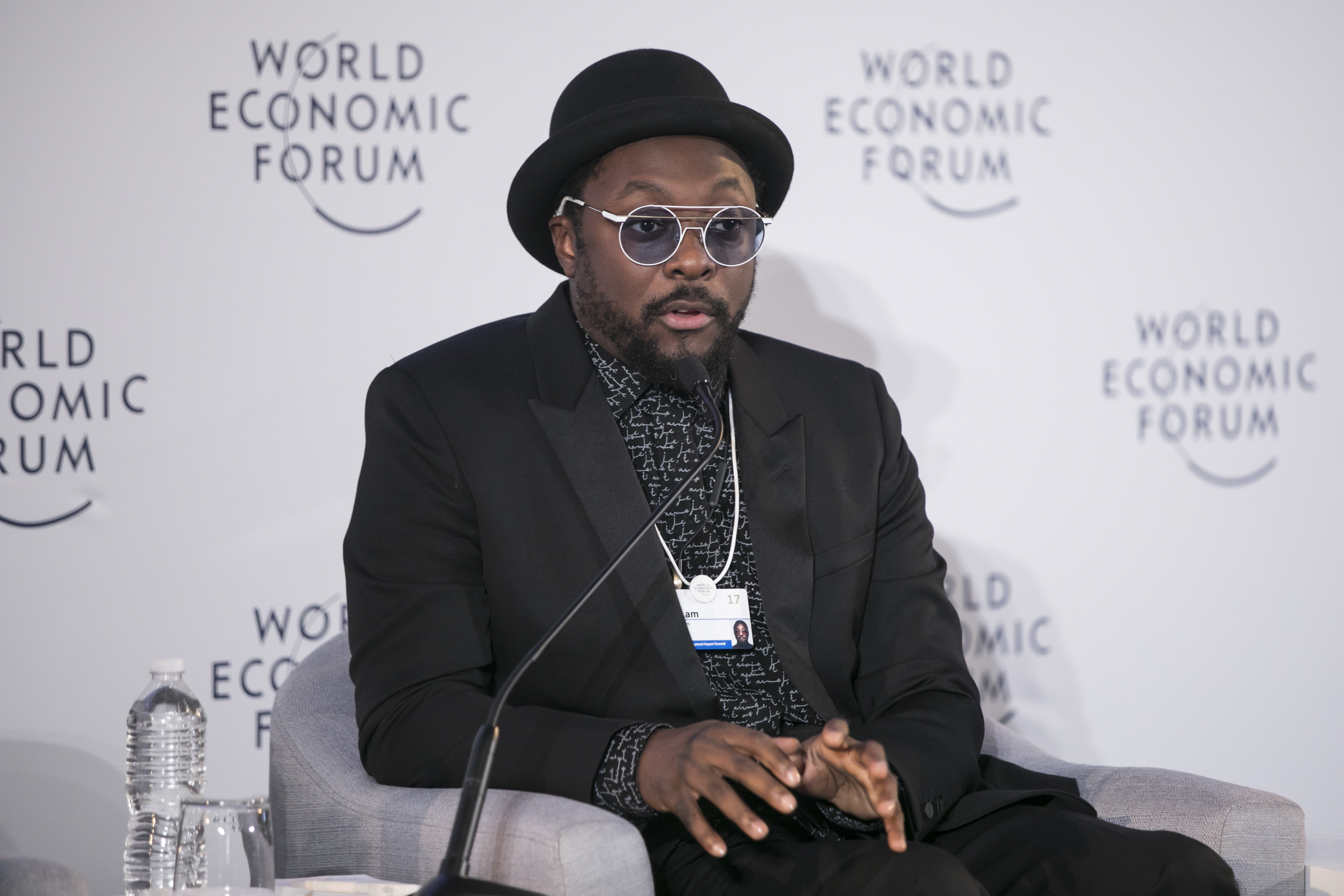The photograph features a well-dressed African American man seated in the center, in front of a logo wall for the World Economic Forum. He has medium dark skin, a full mustache, and a closely cropped beard. He is wearing a black bowler hat and metal round-rimmed glasses. His attire includes a black suit over a black and white patterned button-down shirt, paired with black pants. Around his neck, he wears a name tag on a necklace. 

He is seated in a gray upholstered chair with arms, and a thin microphone boom is positioned near his mouth, suggesting he is speaking to an audience. His arms are bent at the elbows, resting on the chair's arms, and his hands are slightly flexed above his lap, as if emphasizing a point. 

To the lower left corner of the image, there is a small table with a bottle of water and an upside-down glass. The background wall is white, repeatedly displaying the World Economic Forum logo, which consists of the words "World Economic Forum" in black lettering, stacked with each word on a separate line, and a half-circle underline beneath "Forum." The lighting in the image is very good, highlighting the man effectively, giving the impression that he might be an important speaker, possibly a celebrity, musician, or panelist.